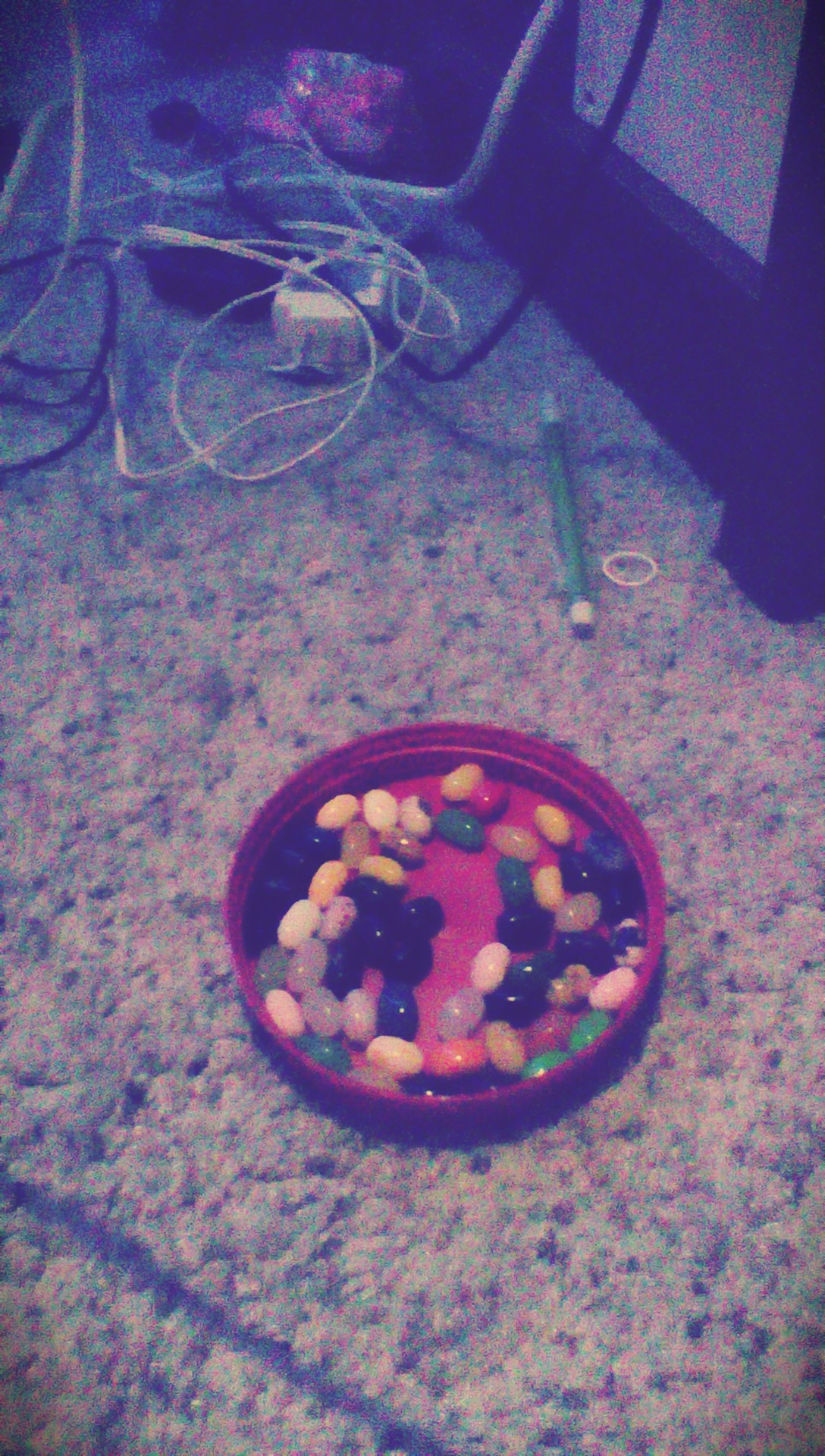An old, grainy photo showcases a shallow red dish, roughly circular in shape, filled with various jelly beans. The jelly beans are vibrant and shiny, featuring an array of colors including blue, multiple shades of green, yellow, white, pink with speckles, red, orange, cream, and translucent yellow. The dish rests on a speckled, sandy-looking surface that could either be a floor or perhaps a table, marked by its green and black polka dots. Behind the dish, there is a green pen or mechanical pencil and to its right, a white rubber band or hair tie can be seen. Several cords, both white and black, extend from the top left of the frame, adding to the cluttered feel of the image. A vague, unidentified red or pink object looms in the distant background. The overall quality of the photo is very low, with notable graininess and coloration issues, likely due to the limitations of an old phone camera.